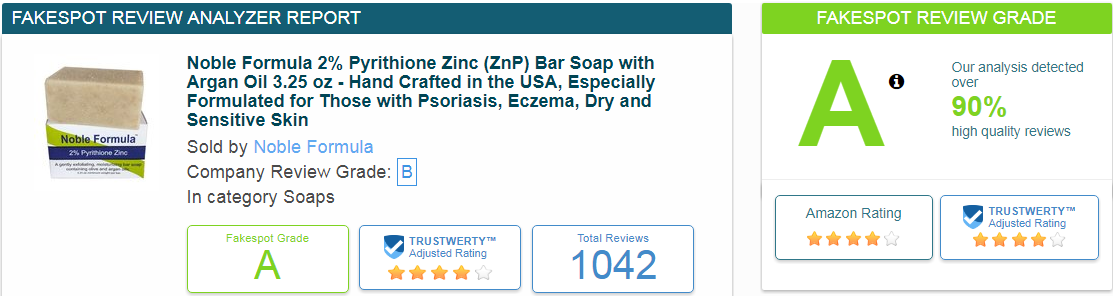Detailed Description Caption:

"Noble Formula 2% Pyrithione Zinc (NP) Bar Soap with Argan Oil (3.25 oz), Handcrafted in the USA. Specially formulated for individuals with psoriasis, eczema, dry, and sensitive skin. The product has a high customer satisfaction rating, achieving an 'A' grade from FakeSpot based on the analysis of numerous reviews, with over 90% being of high quality."